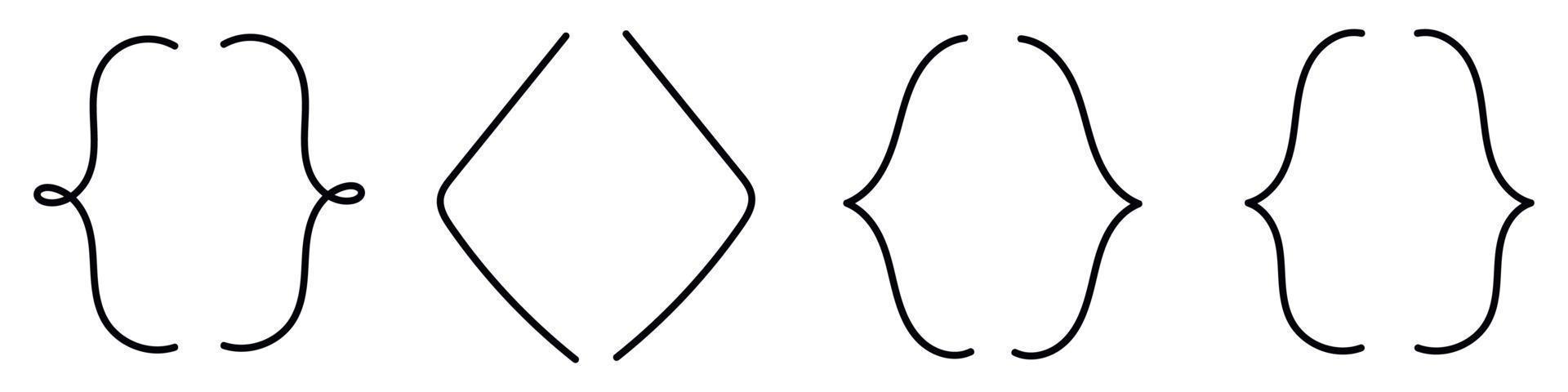The image showcases four distinct groups of shapes, each resembling different styles of brackets or paired lines. Moving from left to right:

1. The first group consists of curved lines that form a pair of curly brackets. These lines have an undulating pattern, starting with a curve at the top, looping inward near the middle, and curving downward at the bottom. Their overall shape can be likened to a stylized set of lips, but with small looped structures in the corners.

2. The second group features triangular brackets, similar to greater-than and less-than signs. These two lines meet at a central point, forming a wide "V" shape, but they do not connect at the top or bottom.

3. The third group presents a pair of lines resembling a tulip shape. The lines are more rounded at the top, curving inward to meet at a sharp point in the middle, before curving outward again.

4. The fourth group is similar to the third, but with subtle differences: the top is flatter, the curve is more pronounced, and the bottom is slightly less rounded, creating a shape that is reminiscent of the previous tulip-like form with a flatter and more angular finish.